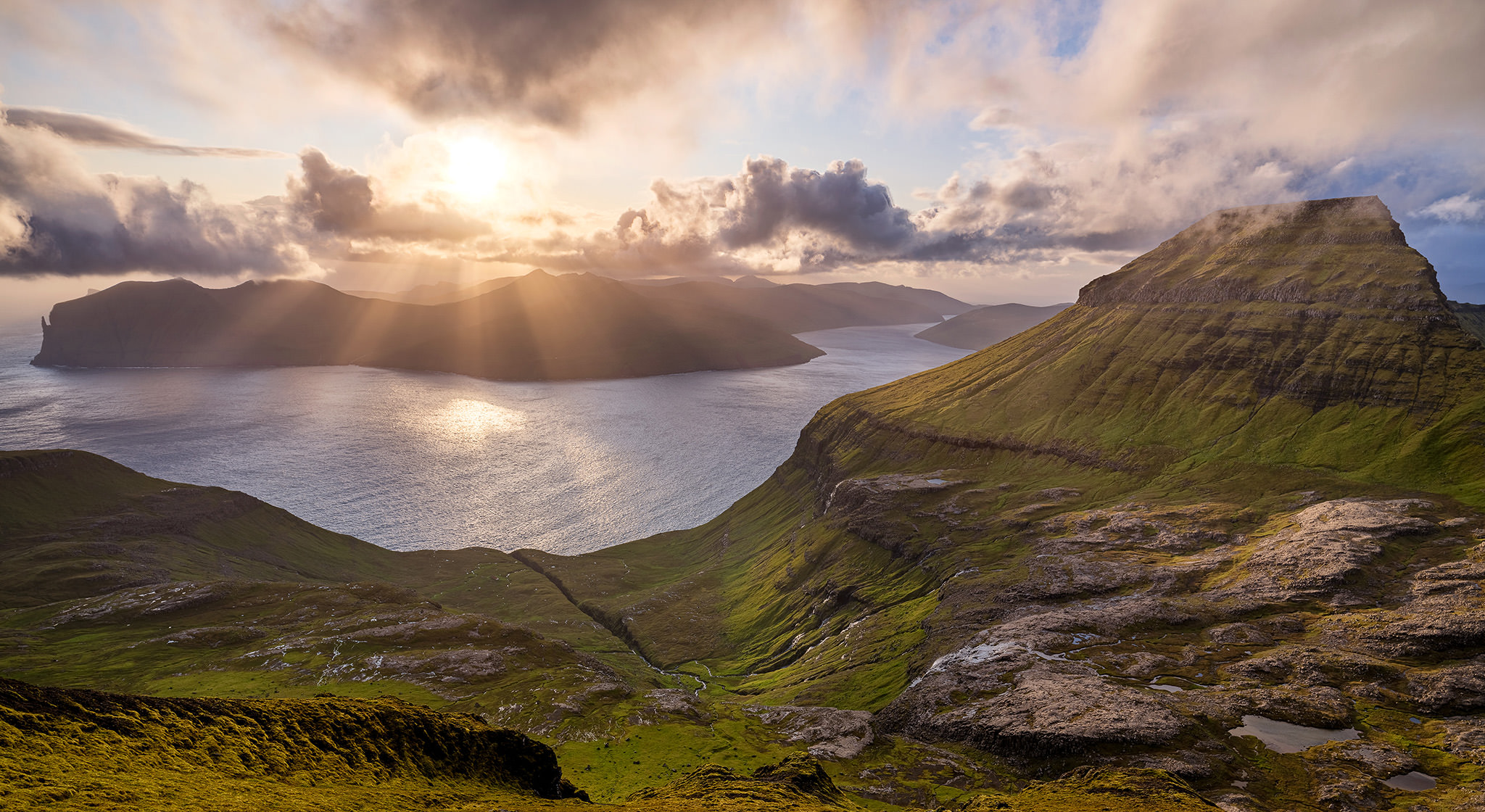This photograph captures a breathtaking, vivid landscape of a mountainous region with lush green hills and grayish rocks adorned with patches of moss. In the foreground, small pools of water are visible amid the rocky terrain. The centerpiece is a towering, verdant mountain, set against the backdrop of a brilliant blue body of water, which extends to a distant island lined with silhouetted mountainous shapes. The sky is an intricate tapestry of blue, white, and dark gray rain clouds, through which the Sun beams its rays, casting a beautiful interplay of light and shadow over the mountains, water, and island. The realistic style of the photograph, devoid of any text, accentuates the natural beauty of this serene, sunlit landscape at either sunrise or sunset, with rippling waves and intricate cloud formations adding depth to the scene.